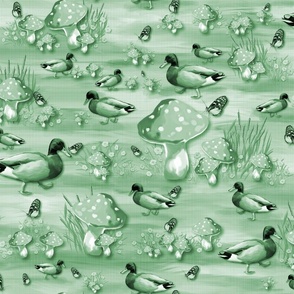This artwork is a detailed illustration that combines a repeating pattern of mushrooms, ducks, and butterflies, all rendered primarily in shades of green. The composition covers the entire canvas, creating a lush, mini garden-like scene. The mushrooms vary in shape and size, featuring the classic triangular tops adorned with polka dots, some accompanied by tufts of grass or elongated leaves. Scattered among these mushrooms are adult and baby ducks, depicted in various poses—some walking left to right and others right to left. Additionally, delicate butterflies are either perched atop the mushrooms or fluttering nearby, enhancing the whimsical, natural feel of the piece. The intricate arrangement of these elements forms a visually rich tapestry that seamlessly repeats throughout the artwork.